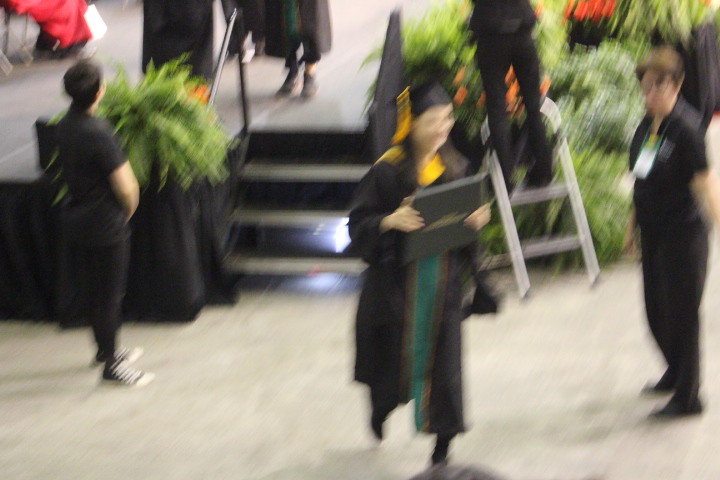In this blurred photograph of what appears to be a college commencement ceremony, a young Caucasian female graduate with long brown hair is captured mid-descent from a black stage adorned with a black curtain. She wears the traditional black cap and gown, accented with a green stripe running down its front. Her cap features a gold stole, and over her shoulders, she drapes a matching gold scarf. She clutches her diploma proudly in front of her. Surrounding her are a couple of individuals dressed in black, one of whom wears a lanyard and appears to be part of the event's staff. To the right of the stage, some lush greenery, including ferns, adds a touch of nature to the scene. A person on a stepladder, likely the event's photographer, captures the moment graduates receive their diplomas. Another graduate, whose legs and lower gown are visible, approaches the stairs. On the far left, seated in a red robe, sits an individual, further adding to the ceremonial atmosphere.